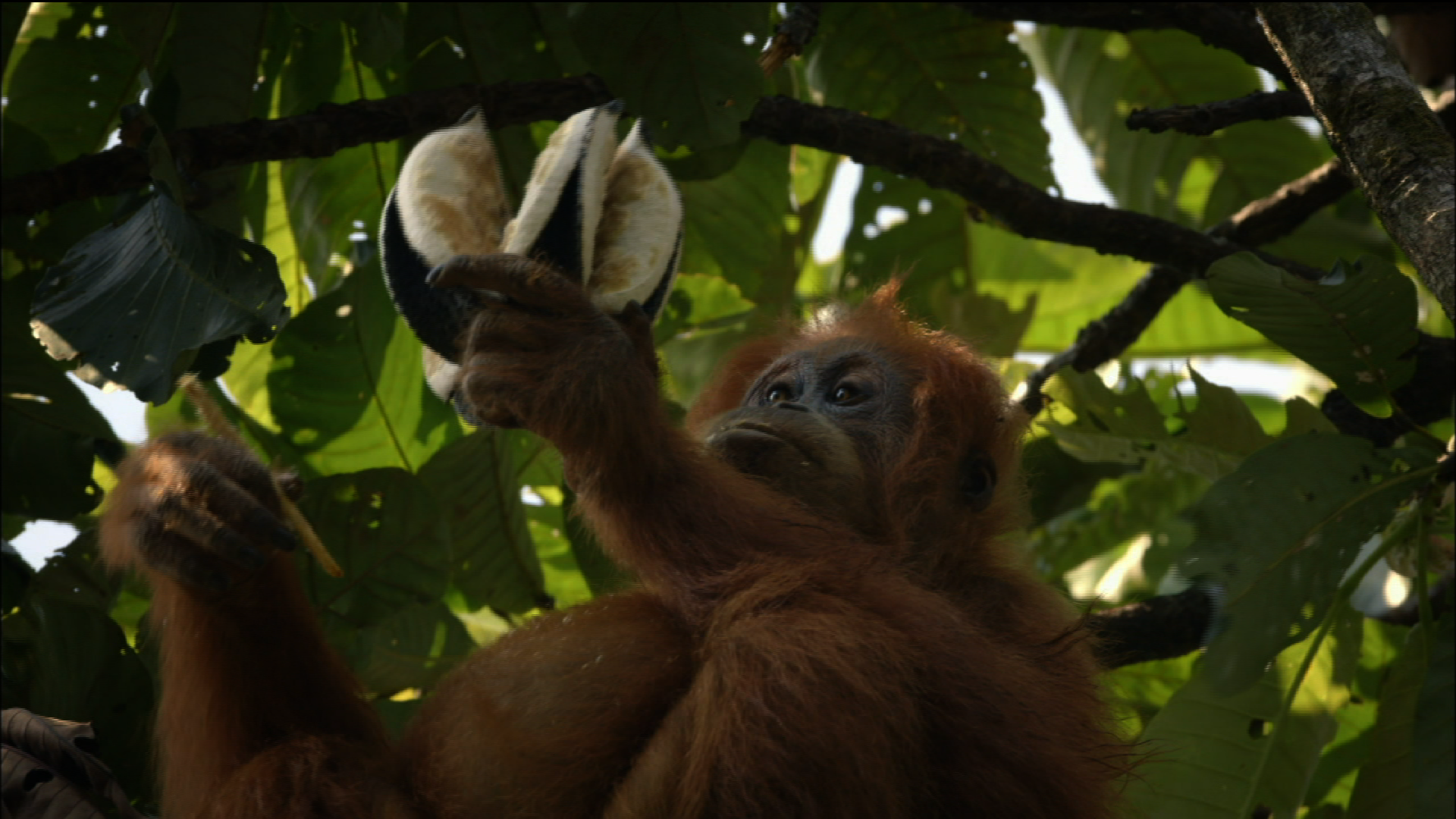This high-definition wildlife photograph captures a detailed scene of a brown-haired baboon perched on a tree branch amidst a lush, tropical landscape. The background is filled with vibrant green leaves and glimpses of the sky, with sun rays filtering through, casting a serene glow on the scene. The baboon, with its distinctive gray face, large dark eyes, and pursed lips, is prominently featured in the lower half of the image. It is seen intently holding a coconut or a similarly colored white and black fruit with one hand, while its other hand grasps a twig for balance. The baboon’s gaze is directed towards the upper left corner, adding a sense of curiosity and engagement to the composition.